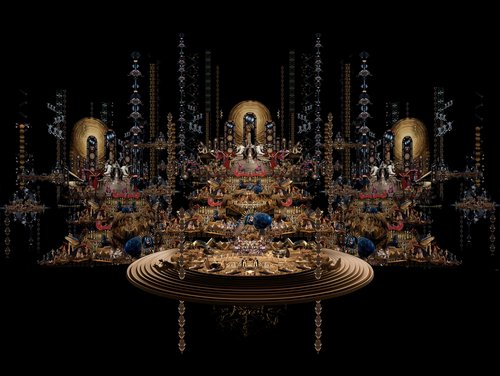The image depicts a mysterious, abstract scene set against a black background. Central to the composition is a broad circular shape that resembles a floor or perhaps a table, adorned with a variety of items, predominantly gold in color but interspersed with hints of blue and red. The circular object is rich with detail and is positioned prominently in the middle, suggesting it is the focal point of the image. Surrounding this main feature are intricate, chain-like elements cascading from the top to the bottom of the image; they vary in color from the dominant gold to dark shades of blue and black.

Additional circular objects are spaced around the center of the image, specifically on the left, middle, and right sides. These elements appear to resemble small, golden waves or ripple patterns. The overall layout suggests a triptych-like structure, with three distinct sections, each containing enigmatic, iconographic obelisk shapes. The central section, being the most elaborate, draws the eye with its intricate design, yet the exact nature and purpose of the items within the circular space remain a captivating mystery.